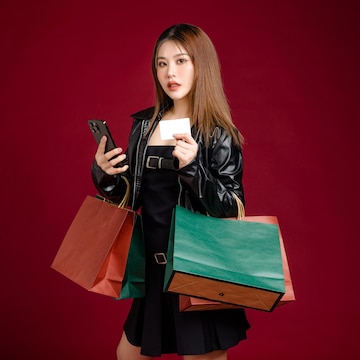The image is a square photograph featuring a stylish woman with Asian features, likely in her 20s or 30s, set against a deep, burgundy red background that subtly lightens towards the center. She stands centrally, facing slightly to the left while looking directly at the camera. Her straight, long brown hair frames her face, embellished with red lipstick. She is dressed in a black leather jacket and a black dress with distinctive belt details across the chest and waist areas. The dress is knee-length.

In her right hand, she holds a black cell phone, while her left hand clutches a small white piece of paper, comparable in size to a business card. Draped over the crook of her elbows are several shopping bags: a red one and partly visible green bag on her left side, and on her right, she carries both a green bag prominently and a red bag partially obscured behind it. The woman exudes a poised and fashionable demeanor in this professionally taken photograph, which offers no visible text.